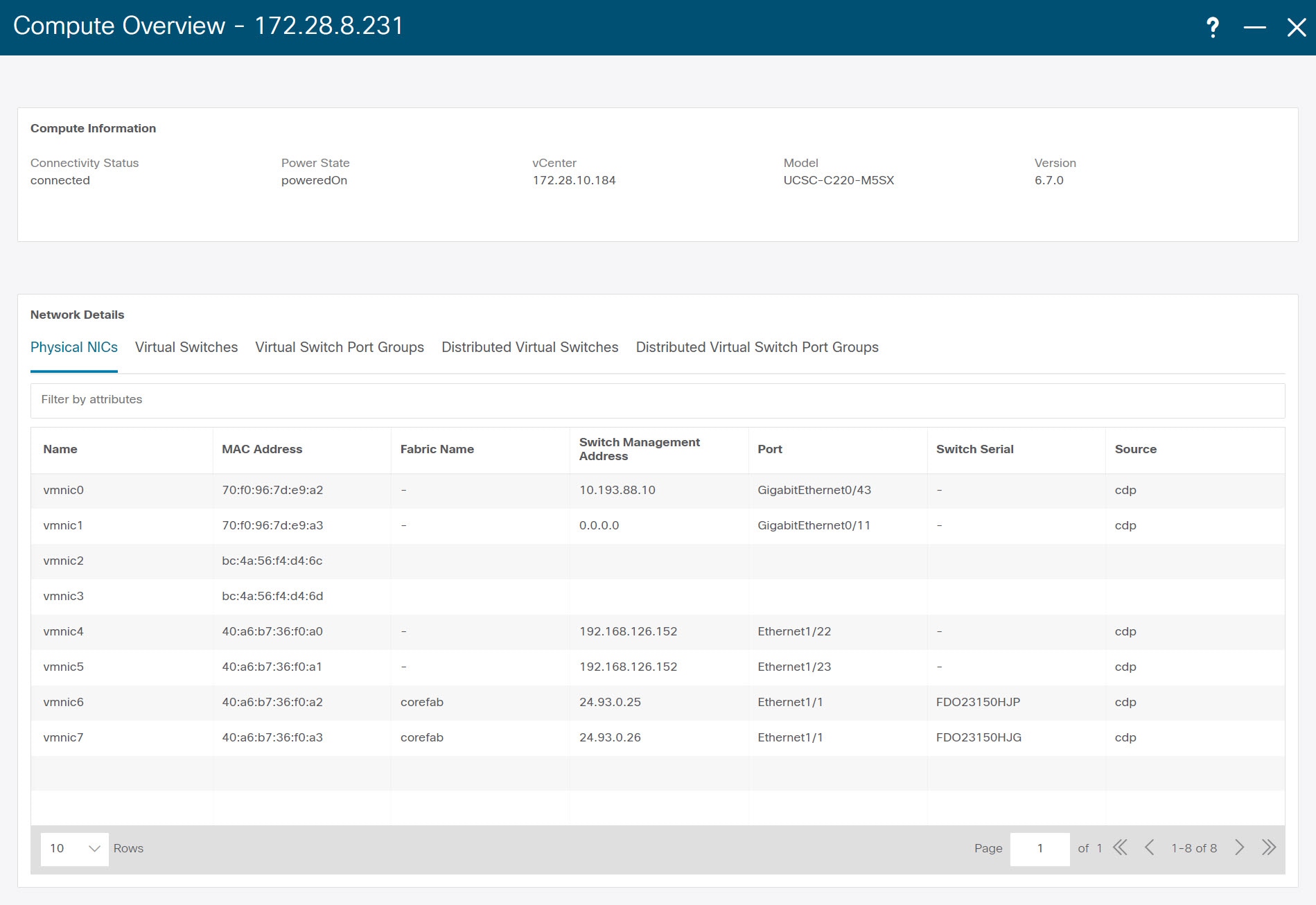At the top of the image, there is a blue rectangle with white text in the top left corner that reads "Compute Overview." Below this, on a gray background, there is a white rectangle with the heading "Compute Information." Under this heading, various statuses are listed including "Connectivity Status," which is marked as "Connected," and "Power State," which is marked as "Power On." There is also a section labeled "Data Center" with associated numbers, followed by sections indicating "Model," with corresponding letters and numbers, and "Version."

Further down, another white rectangle is divided into alternating white and gray lines. This section contains headers such as "Physical NICs," "Virtual Switches," "Virtual Switch Port Groups," "Distributed Virtual Switches," and "Distributed Virtual Switch Port Groups," extending from left to right. 

Under these headers, columns are organized from left to right displaying information such as "Name," "MAC Address," "Fabric Name," "Switch Management Address," "Port," "Switch Serial," and "Source." The gray and white background pattern continues down this section, with each row populated by corresponding data such as names and MAC addresses under their respective columns.